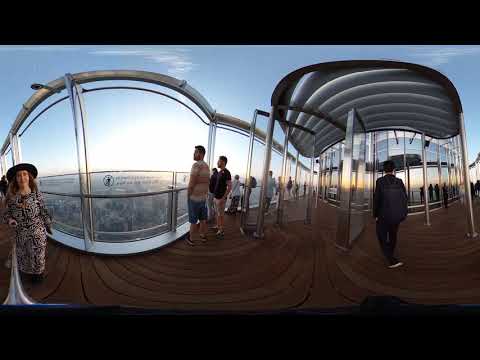The image is a bright panoramic photo taken from a selfie stick atop a high structure, possibly a skyscraper or a bridge, with a wooden floor. The ground features upside-down rainbow stripes and three loops. On the left, a smiling woman in a black and white patterned dress and a black wide-brimmed hat is holding the selfie stick. Behind her, there is a rounded-edge glass barrier with a metal bar across, with an oval semi-circle metal arch above it extending towards the horizon. Metal poles are scattered around. The sky is a clear blue, enhancing the bright atmosphere. On the right side, a person dressed in black with a backpack walks along. The background reveals a cityscape viewed through glass walls, reflecting the sun, with numerous people standing and walking on the elevated walkway, gazing into the distance.